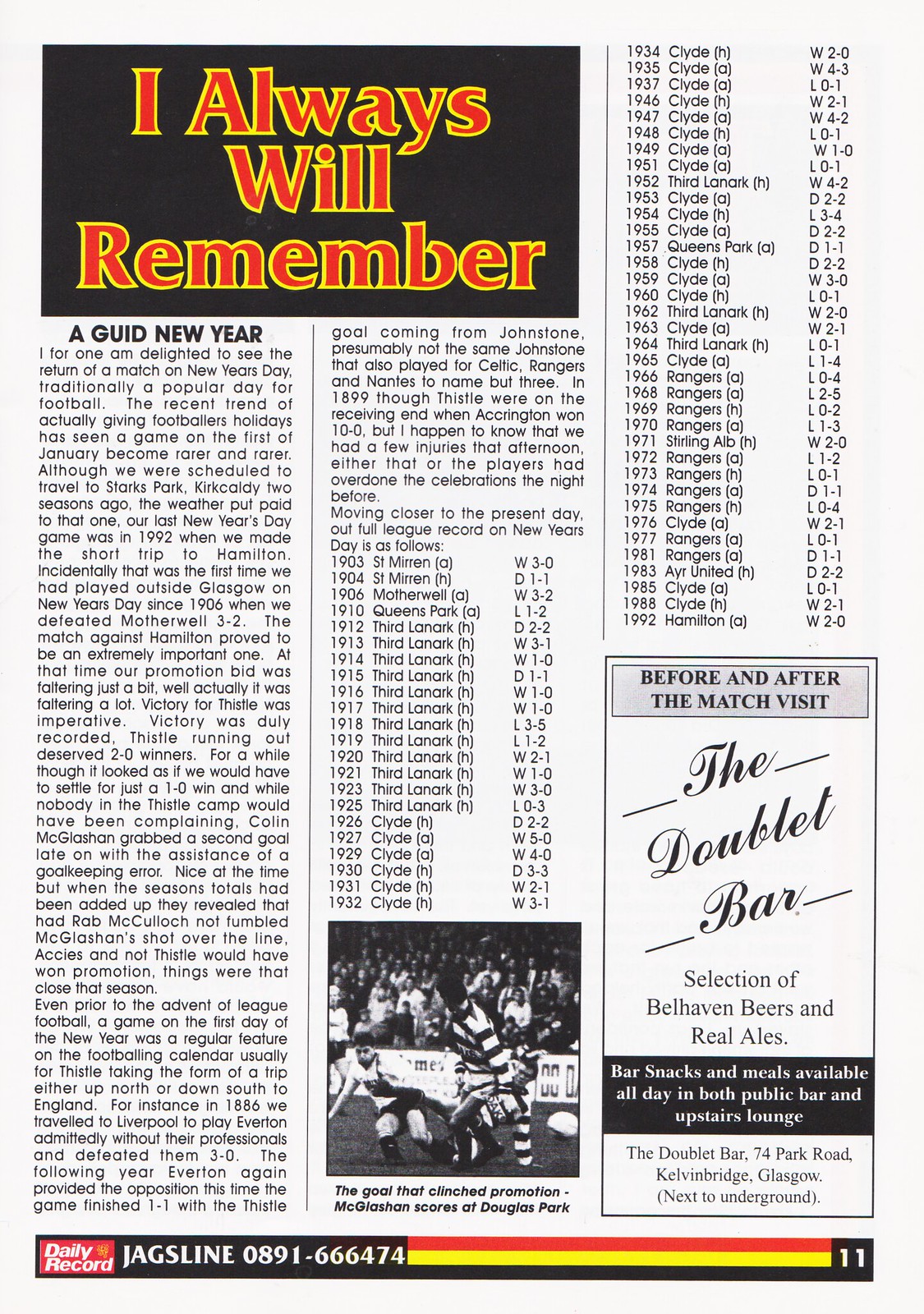The image depicts a page from a newspaper featuring an article about the traditions of New Year's Day football. Prominently displayed in the top left corner is a striking black rectangle with the words "I always will remember" in red letters outlined in yellow. This title captures the essence of the nostalgic piece.

Below the heading, the article discusses the excitement of returning football matches on New Year's Day, a day traditionally celebrated with popular football games. The author expresses delight at this resurgence, noting that the trend of granting footballers holidays had made January 1st matches increasingly rare. The article reminisces about past matches, mentioning an attempted but weather-cancelled trip to Starks Park, Kirkcaldy, two seasons ago, and the last played New Year's Day game in 1992 against Hamilton.

Additionally, the page features an advertisement highlighting the Doublet Bar, which offers a selection of Bellhaven beers and real ales, alongside bar snacks and meals available throughout the day. It provides the bar's address and contact details, emphasizing a welcoming atmosphere for football fans before and after the match. The bottom section also lists scores and winners from previous New Year's Day games.